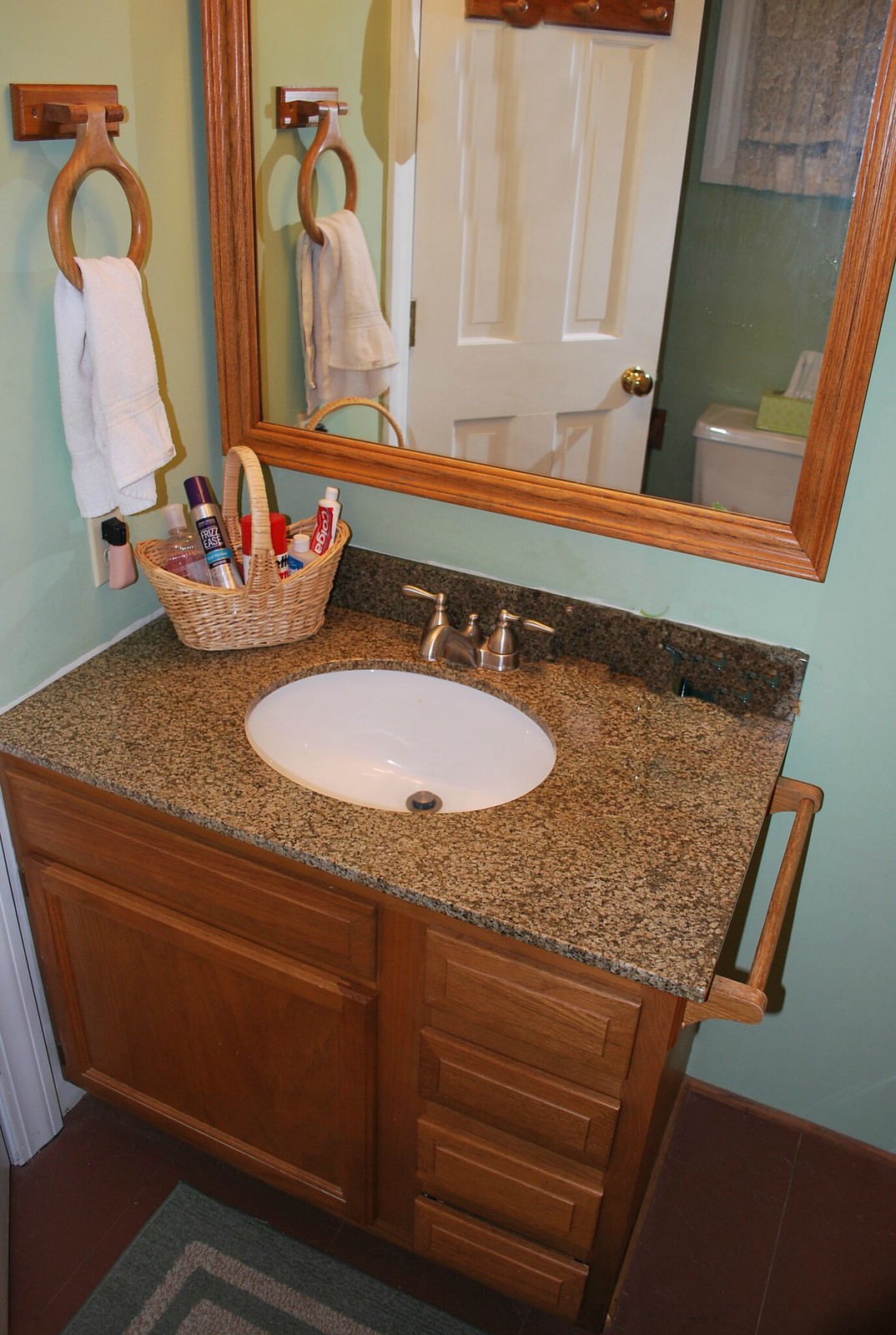This photograph showcases the sink area of a meticulously designed bathroom. The white sink is conveniently placed in a corner where two green-painted walls meet. Above the sink hangs a large mirror with a wooden frame, reflecting a toilet located across the room and a slightly ajar white door. The countertop around the sink features a white and gray mottled design, complemented by silver fixtures including separate handles for hot and cold water. 

On the left side of the counter, a wooden towel ring attached to the wall holds a neatly hanging towel. A basket sits on the upper left side of the countertop, brimming with various bathroom essentials, including a tube of Colgate toothpaste and several other squat containers. Below the sink, multiple drawers and a larger cabinet offer ample storage space. 

To the right of the sink setup, a wooden towel rack is affixed to the wall, contributing to the room's cohesive decor. The wooden floor beneath the sink is adorned with a green and white rug, adding a touch of comfort and color. The entire setup blends practicality with aesthetic appeal, creating a welcoming and functional bathroom space.